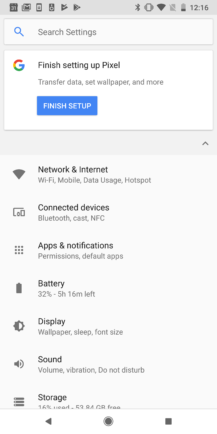A screenshot of the "Settings" page on an Android Pixel phone is displayed. At the top of the screen, a prompt reads, "Finish setting up Pixel: Transfer data, set wallpaper, and more," accompanied by a blue "Finish setup" button. Above this prompt is a search bar for navigating the settings. Below the prompt, the general settings categories are listed with their respective icons and brief descriptions. These include:

- **Network & Internet**: Wi-Fi, mobile data usage, hotspot
- **Connected Devices**
- **Apps & Notifications**
- **Battery**: 32%, 5 hours 16 minutes left
- **Display**
- **Sound**
- **Storage**: 16% used, 53.84 GB free

The remainder of the categories trails off but continues down the page. The notification area above shows ongoing activity. The background of the settings page is a light gray, creating a clean and organized look. This suggests the phone has recently been set up, but some configuration steps were skipped, prompting the device to remind the user to complete setup for an optimized experience.